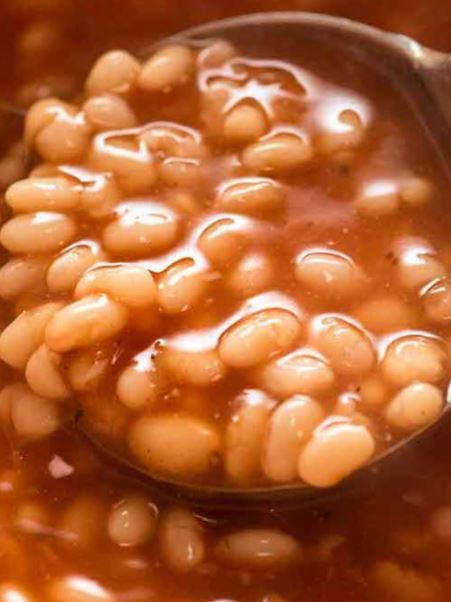The image depicts a very close-up view of a large wooden spoon, prominently positioned and almost overflowing with a hearty scoop of white kidney beans enveloped in a thick, brownish-orange, sauce-like liquid. The spoon, which is dark brownish-red in color, occupies a majority of the frame, suggesting it is dipping into an unseen larger container filled with the same bean mixture. The beans themselves are oval to crescent-shaped, meticulously coated in the rich, reddish-brown sauce that fills the entire background. The photograph is vertically rectangular and emphasizes the intricate details and textures of the beans and sauce, giving an impression reminiscent of a traditional bean soup or saucy beans.